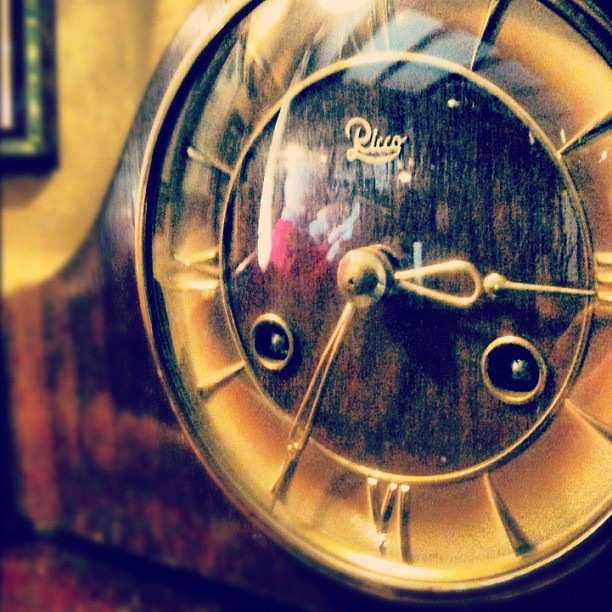The image showcases an elegant golden clock with a black center, prominently featuring gold Roman numerals. Reflected in the clock's glossy surface, an older individual appears to be reading a book or newspaper, suggesting a calm, homey atmosphere. The scene likely takes place in a living area, evidenced by a black picture frame hanging on a yellow wall and glimpses of brown wooden furniture. The clock, centrally positioned, serves as the focal point of the composition, dominating most of the image space.